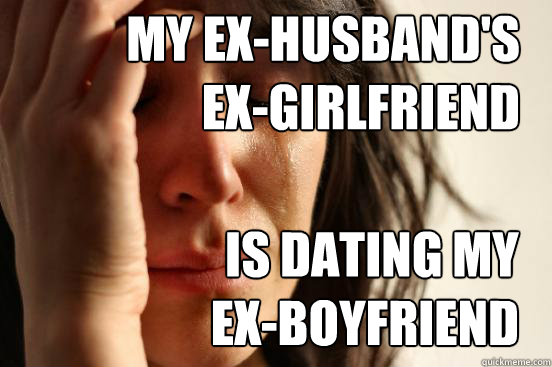In this image, a muscular male wrestler is positioned on all fours on a large bed in what appears to be a bedroom setting. The man has a bald head with a smattering of hair toward the back, and a well-maintained salt-and-pepper stubble beard. He sports a distinctive tattoo on his upper right shoulder and is nearly nude, wearing only a black thong. His chest and legs are covered in hair, with his legs showing a slight tan.

The bed itself is adorned with a camouflage-patterned blanket in shades of red, white, black, and gray, resembling a military camo design. Surrounding the man are black and white leather pillows with white piping. The bed features a dark brown wooden headboard, flanked by two tall, cherry wood bedposts. The background consists of a dark gray wall, which might be brick, providing a stark contrast to the bed's elements.

Below, near the bottom of the image, two white electrical outlets are visible on either side of the bed, indicating a modern setting. The scene is well-lit, suggesting that this photograph could be part of a professional set.